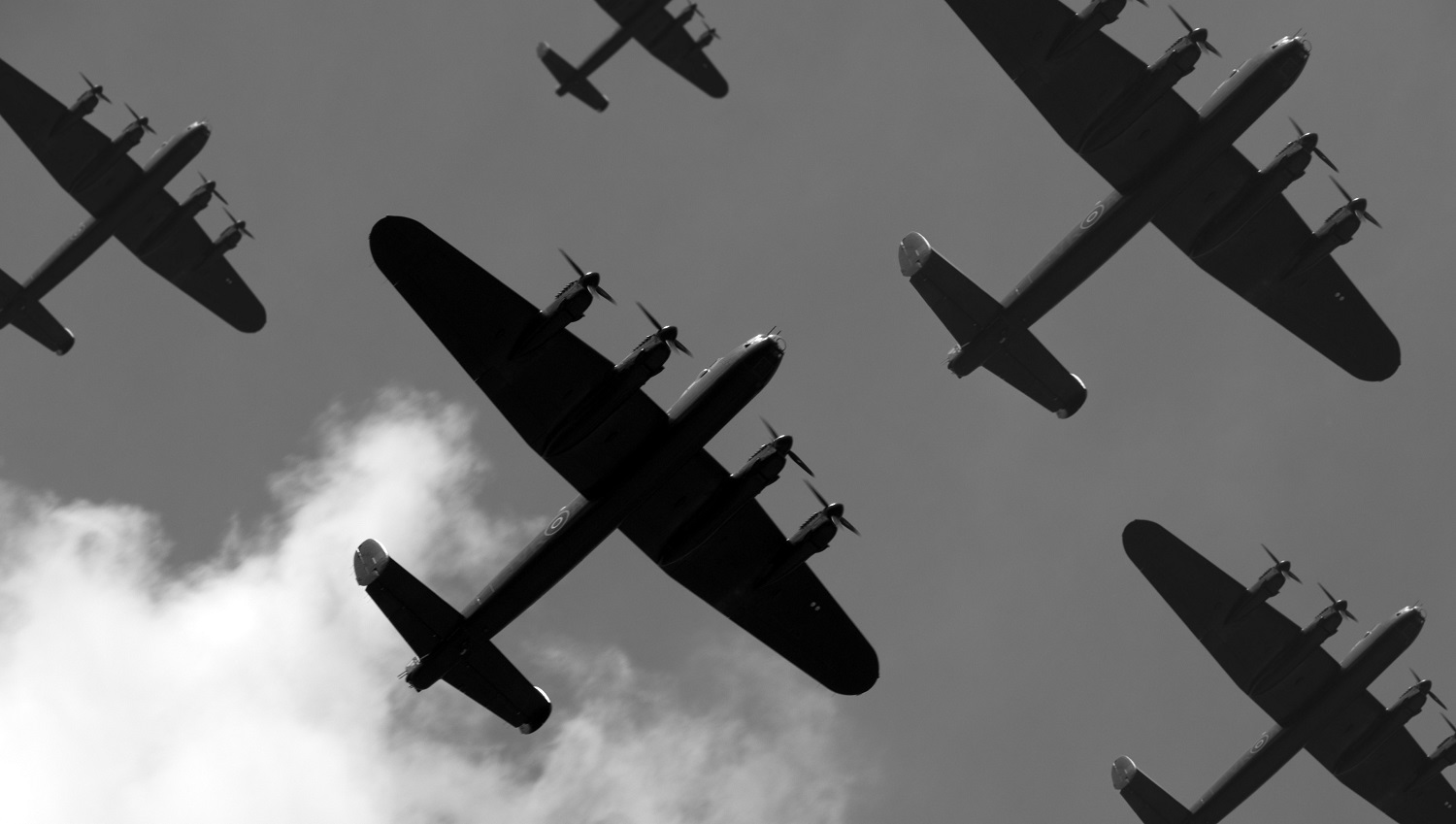This black and white photograph, horizontally oriented, captures a dramatic aerial view of five vintage fighter planes set against a solid medium gray sky. The planes are ascending diagonally towards the top right corner of the image, adding a dynamic sense of movement. The lower left-hand corner features a cluster of puffy white clouds, contrasting with the otherwise uniform sky. 

The central plane, viewed from its underside, reveals detailed features: twin propellers on each wing, and a distinctive tail and wing structure. Some planes are partially cropped, including one in the upper left with its left wing and tail cut off, another in the lower right missing part of its right wing and tail, and a third in a central position with part of its left wing cut off. A fourth plane is higher up and further away, giving a sense of depth to the formation. The overall composition and technical aspects of the planes—characterized by black and gray undersides against the lighter sky—highlight the vintage, military nature of these aircraft. The photograph’s detailed rendering of the planes’ propellers, each with four blades, two on each wing, enhances the historic feel.